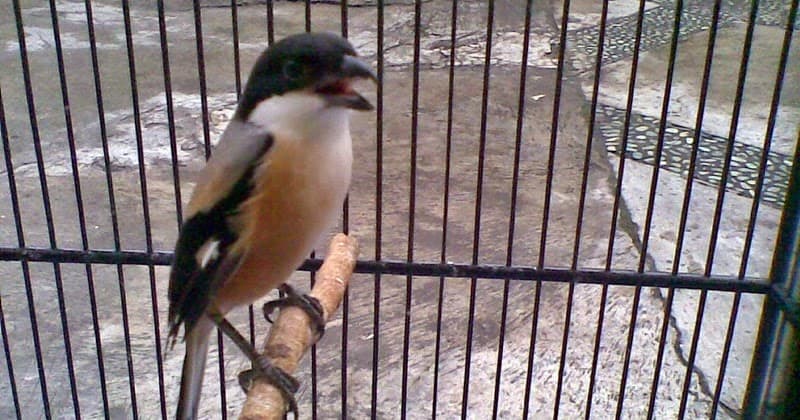The image captures a small songbird perched inside a cage, offering a perspective as if viewed from within. The bird is positioned toward the center left of the photo, gripping a sturdy branch or stick that's part of the cage setup. Its head is black, with an open beak, revealing a glint of a dark eye. The bird's feathers display a striking color palette: a light yellow neck transitions to an orangish-brown belly, while its wings feature a gradient from white and orangish-brown to black with a noticeable white spot. The underside of its tail feathers is white, whereas the upper side, turned away from the viewer, along with the rest of the tail, remains unseen. The cage's vertical bars frame the bird, and through them, you can glimpse an exterior ground surface that appears to be a mix of dirt, cement, and stone or tile, evoking the feeling of being in an enclosed environment, possibly at a zoo.